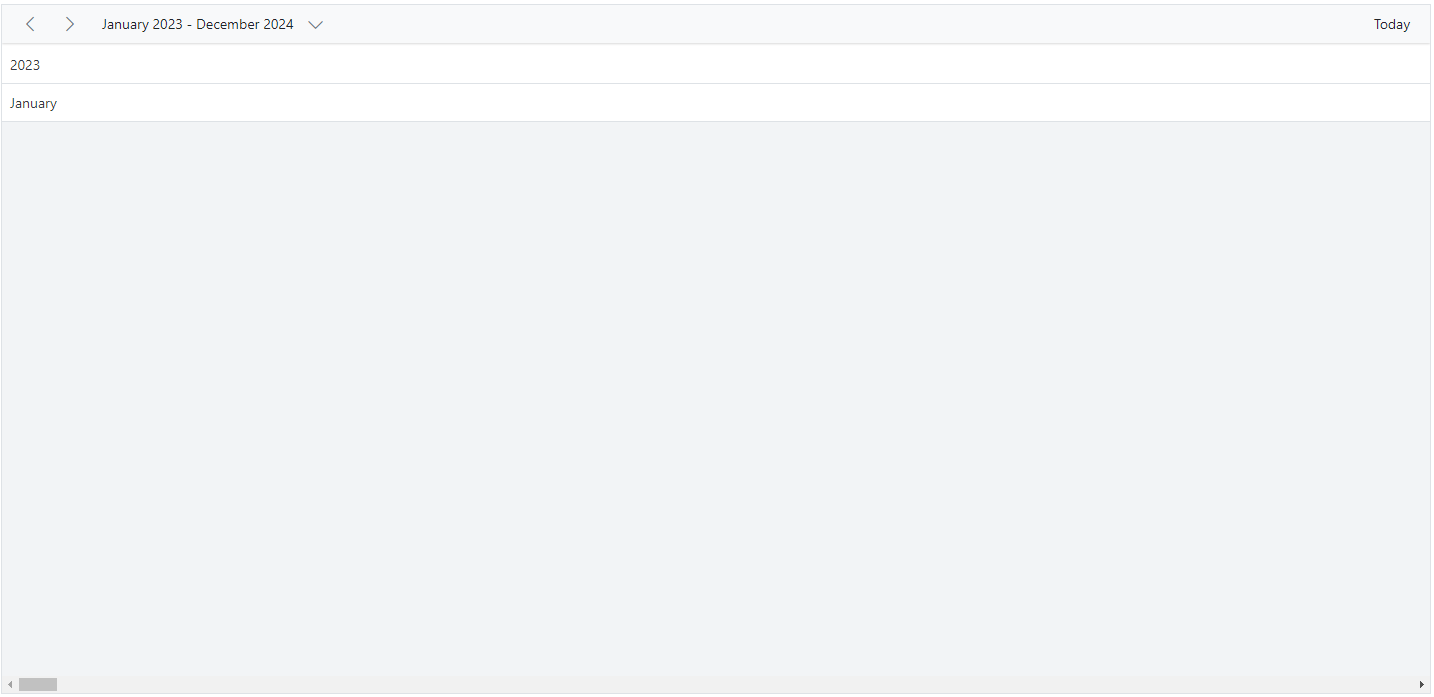The image is a minimalist digital interface, likely a calendar or email scheduling tool, dominated by shades of white and gray. At the top-left corner, there are two navigation arrows (left and right). Adjacent to these arrows is a date range selector specifying "January 2023 to December 2024," accompanied by a drop-down menu. On the far right of the top row is a button labeled "Today." Directly below this, the second row features only the year "2023," leaving a considerable amount of blank space. The third row contains the label "January."

Beneath the "January" label is a large, empty text box that occupies approximately 70-80% of the image, shaded in gray, offering no further content within it. At the bottom of the image, a horizontal slider indicates that this view is just a portion of a larger file. Adjusting the slider to the right would potentially reveal additional information or content, highlighting that this is only a snapshot of a more extensive dataset or interface.